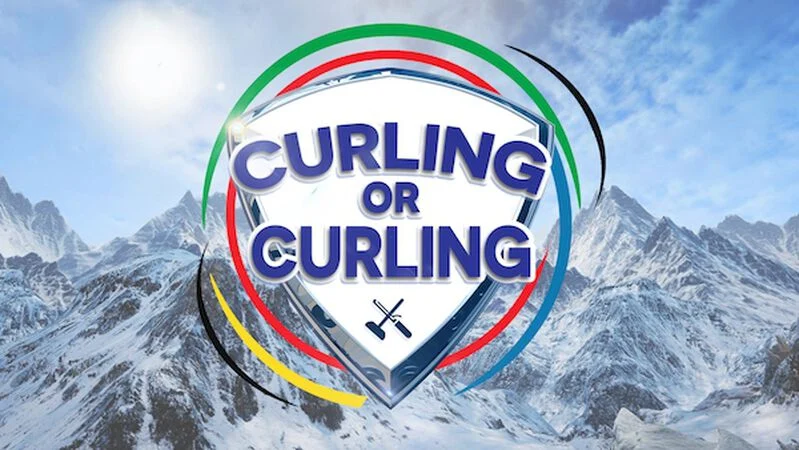The image depicts a poster associated with the Olympic Games, featuring a central white shield emblem outlined in silver and blue hues. The word "curling" is prominently displayed in blue letters within the shield. Surrounding the shield are semi-circular swoosh patterns in various colors—green, red, blue, yellow, and black—symbolizing the Olympic spirit. Inside the shield, below the text, are tiny black silhouettes of curling equipment, likely representing a curling broom and stone. The background showcases a picturesque snowy mountainous region under a blend of a hazy blue sky, clouds, and partial sunlight in the upper left corner, evoking the chilly ambiance of winter sports.